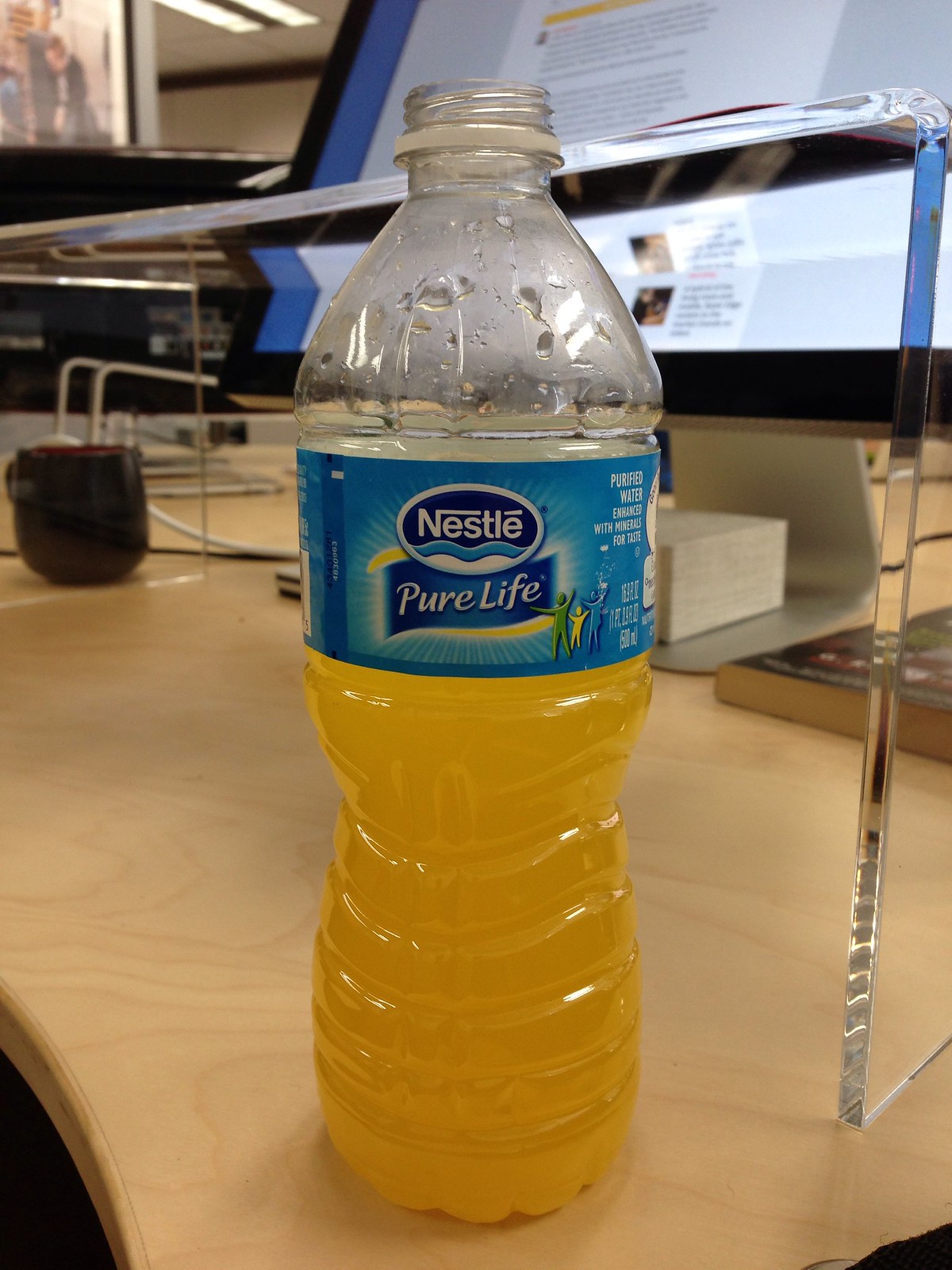This is a high-quality photograph of a desk setup, possibly an office cubicle. Dominating the scene is a Nestle Pure Life water bottle, prominently displaying its white, blue, and dark blue label. The cap is off, and the bottle contains a bright yellow-orange liquid, suggesting the original water has been replaced with a flavored drink. It rests on a light beige, wood-toned desk. To the left of the water bottle, a black coffee mug sits, potentially holding tea. 

In the background, to the right of the bottle, a large, flat computer monitor displays a white image with black text, indicating some work or reading is in progress. Additional details enhancing the office atmosphere include black and white cords on the table and a black object resembling a book next to the bottle. Behind the monitor, a translucent object and a small wooden box are visible beneath it, implying organizational items often found in office spaces. 

A family photo frame and a cubicle divider are slightly visible to the left, reinforcing the office or cubicle setting. Overhead, the ceiling features fluorescent lighting, aligning with a typical office environment.